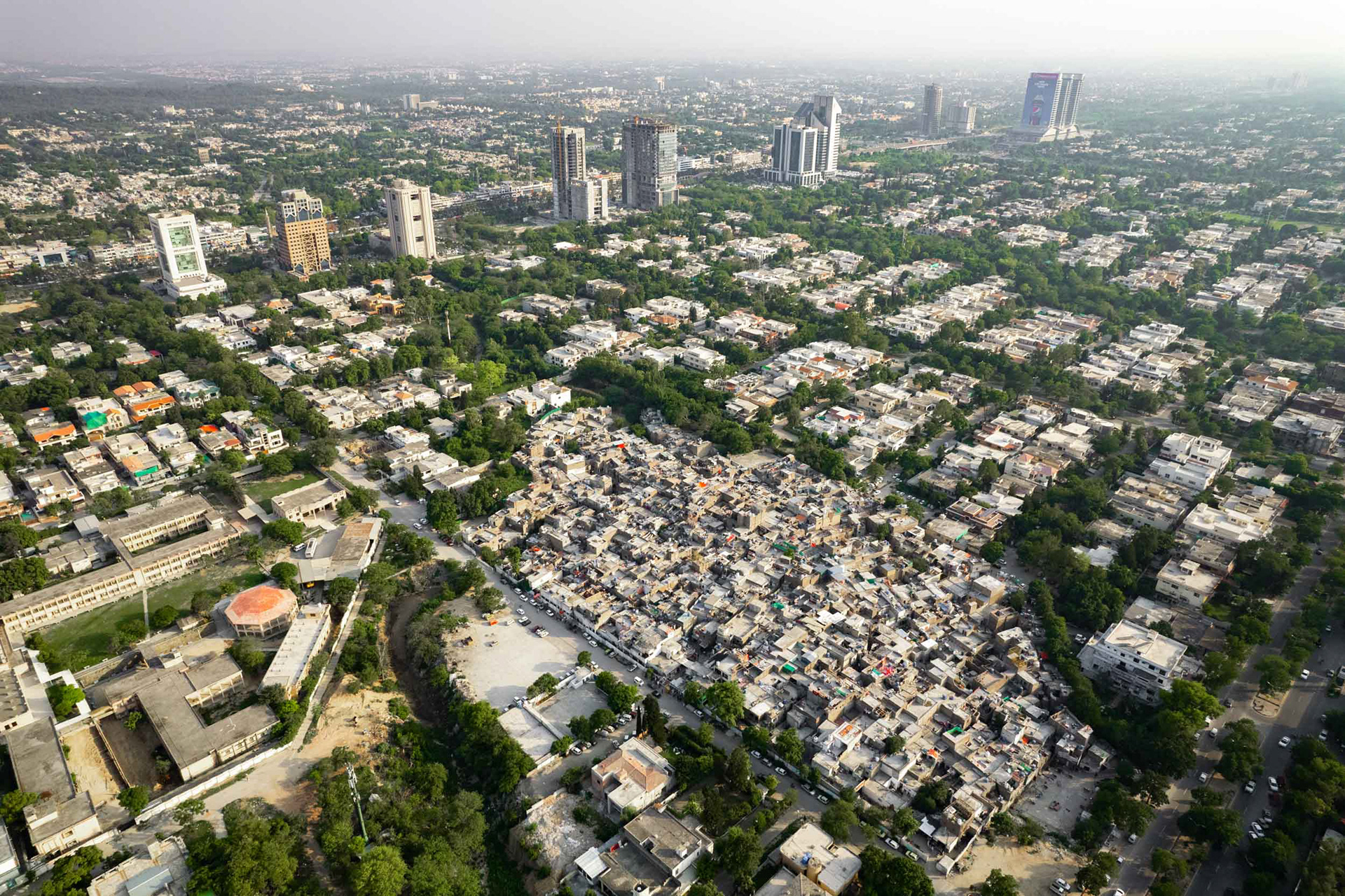This aerial photograph, likely taken from a low-flying aircraft a few hundred feet above the ground, showcases a sprawling urban landscape on a cloudy day. The foreground is dominated by a densely populated area with numerous homes, buildings, and cars clustered together, presenting a slightly chaotic appearance that might indicate a slum or highly congested neighborhood. Surrounding this central area, the city sprawls out in every direction, revealing a mixture of smaller structures, streets, and patches of greenery. About a fourth to two-thirds up the image, a series of high-rise buildings, approximately 20 to 25 stories tall, breaks the skyline, standing in various shades of gray and possibly serving as apartments or office buildings. These skyscrapers line a major street, adding a vertical dimension to the predominantly horizontal sprawl below. The photo, set in landscape orientation, captures a slice of the city's vast and diverse urban fabric, blending dense habitation, commercial zones, and verdant spaces under a largely obscured, cloudy sky.